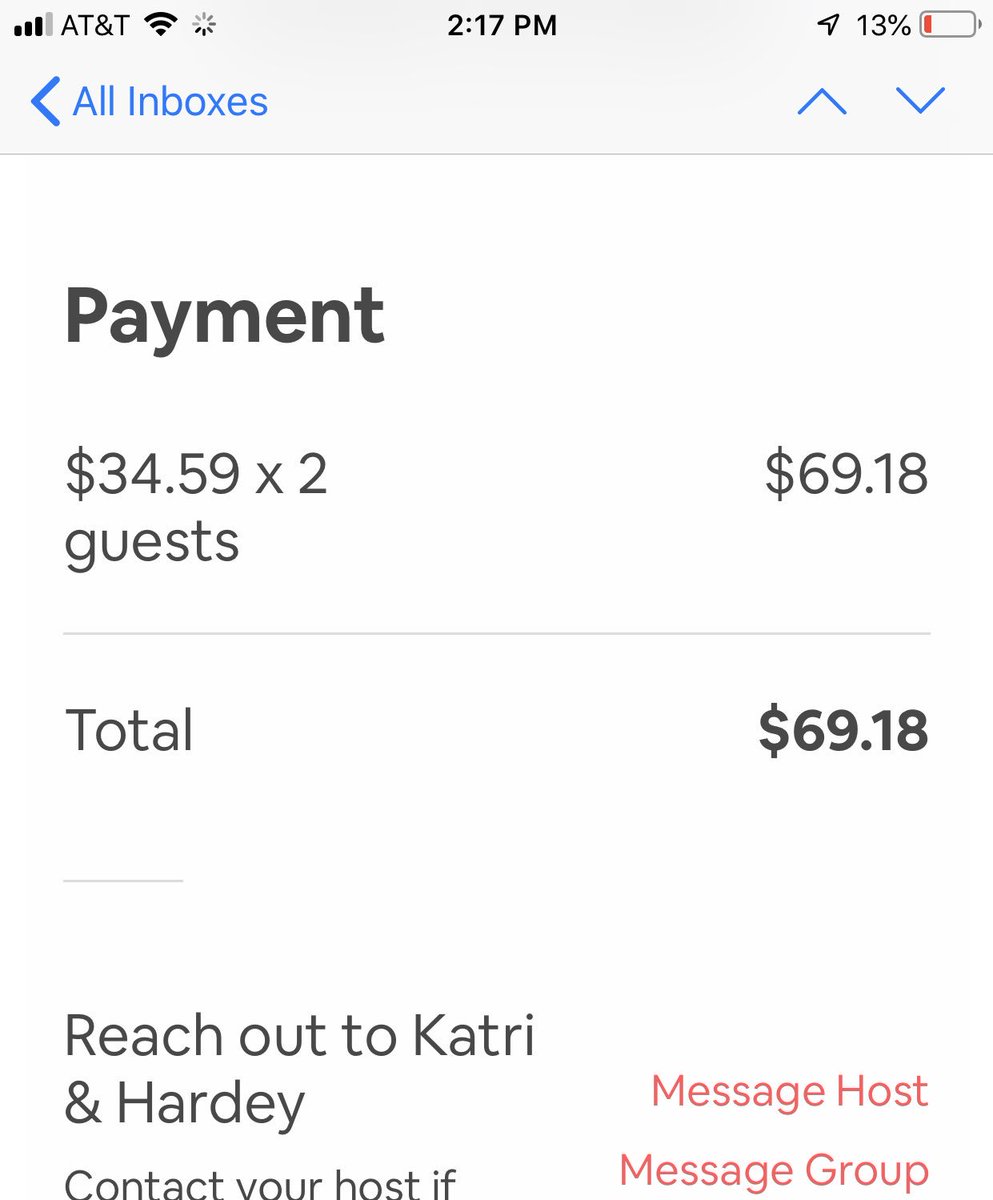The screen displays various indicators and information:

- At the top left, the signal strength indicator shows 3 bars next to the AT&T carrier label.
- Adjacent to it, there is the Wi-Fi strength icon resembling a stylized Walmart flower, indicating a signal strength of 217.
- The battery icon to the right shows a 13% charge.

Below these status icons, the main content is as follows:

- A header reading "All inboxes" in bold, accompanied by a blue left arrow icon.
- Below this header, a section titled "Payment" showing the amount 34.59 multiplied by 2, resulting in 69.18 displayed to the right.
- Directly under these numbers, the screen shows "Total" followed by the sum 69.18, with the total amount highlighted in a slightly larger and bolder font.

At the bottom, there's a message prompting action: "Reach out to Catri in Hardy." It advises the user to contact their host if needed. 

- Below this message, in red, are two call-to-action buttons: "Message Host" and "Message Group."